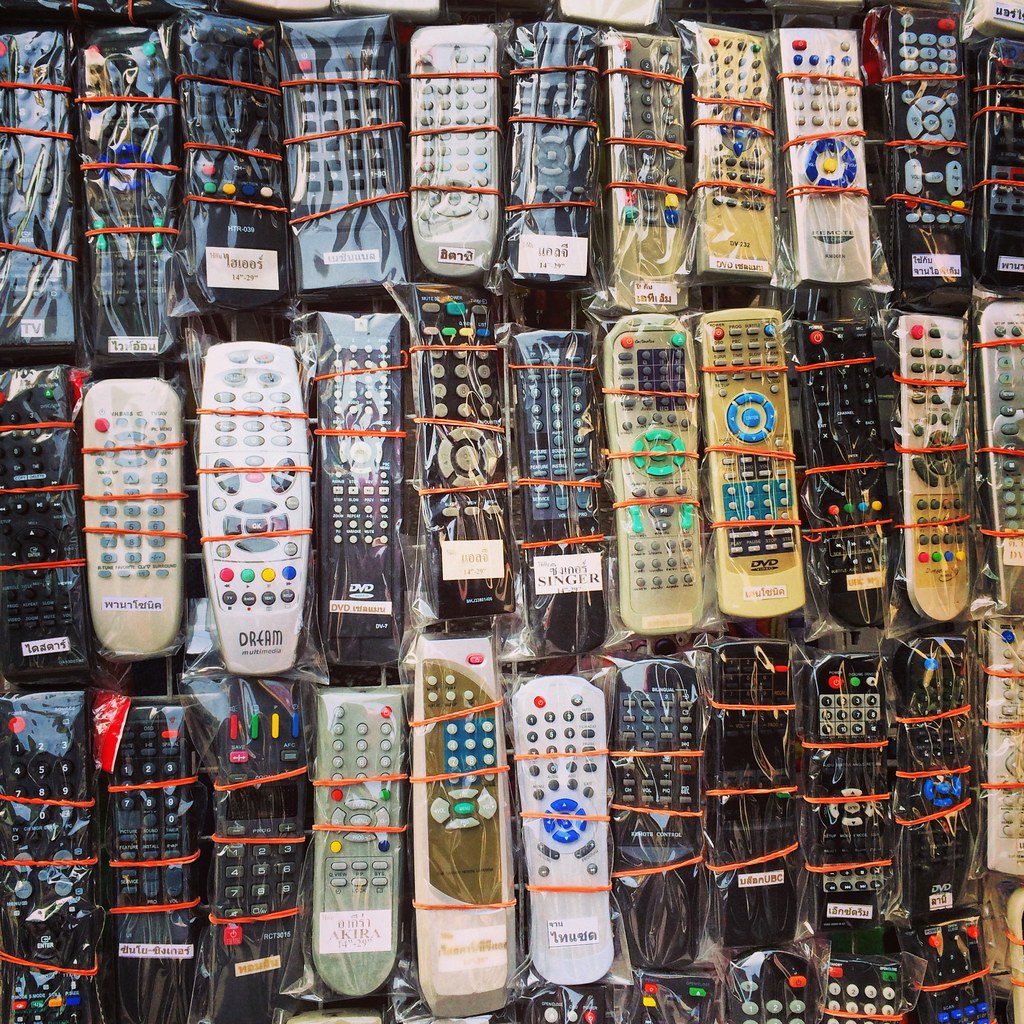This photograph captures a structured display of remote controls, likely set up for sale, possibly at a secondhand store. The image reveals four rows, although only three are fully visible while the fourth is partially cut off at the bottom. Each remote is individually wrapped in clear plastic and secured with three orange rubber bands. The plastic-wrapped devices are of varying colors, including predominantly black, silver, white, gray, beige, and even gold. The buttons on these remotes also differ in color, featuring hues like blue, green, gray, black, navy, and rainbow colors—red, yellow, green, and blue. Many remotes bear labels at the bottom, some of which are in a language that appears to be Hebrew. The brands mentioned include Singer, Akira, and Dream, indicating a diverse assortment of manufacturers. The overall condition of the remotes ranges from well-used and somewhat dirty to newer-looking units. Each remote seems tailored for different devices, such as televisions, DVD players, and VCRs, suggesting a wide variety of products for prospective buyers.